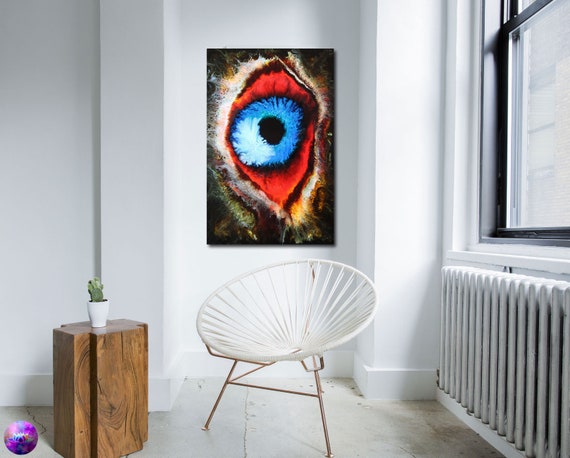This image captures a cozy, modern corner of an urban apartment, possibly located in a city like New York. The focal point is a distinctive, contemporary chair with a metal base and three thin, bronze-colored legs. The seat is designed with a circular, half-clam shape formed by taut ropes or slings that stretch when seated upon, creating a comfortable and visually intriguing form. The chair is accompanied by a minimalist side table made from a carved block of wood with clean, straight edges, which holds a small cactus in a sleek white pot.

Adjacent to this seating area is a classic, white radiator positioned beneath a window that offers a view of another city building. The walls of the room are painted a pristine white, providing a stark, clean backdrop. Hanging on the wall behind the chair is a striking, vertically oriented piece of art featuring a highly stylized eye. The eye's iris is an intense, vibrant blue, surrounded by a red sclera and a white, fuzzy eyelash area, creating a dramatic and modern visual impact. The floor appears to be either whitewashed wood or concrete with distinct texture and perhaps minor imperfections, adding to the urban aesthetic of the space. This inviting nook offers a serene and fashionable retreat for reading or relaxation.